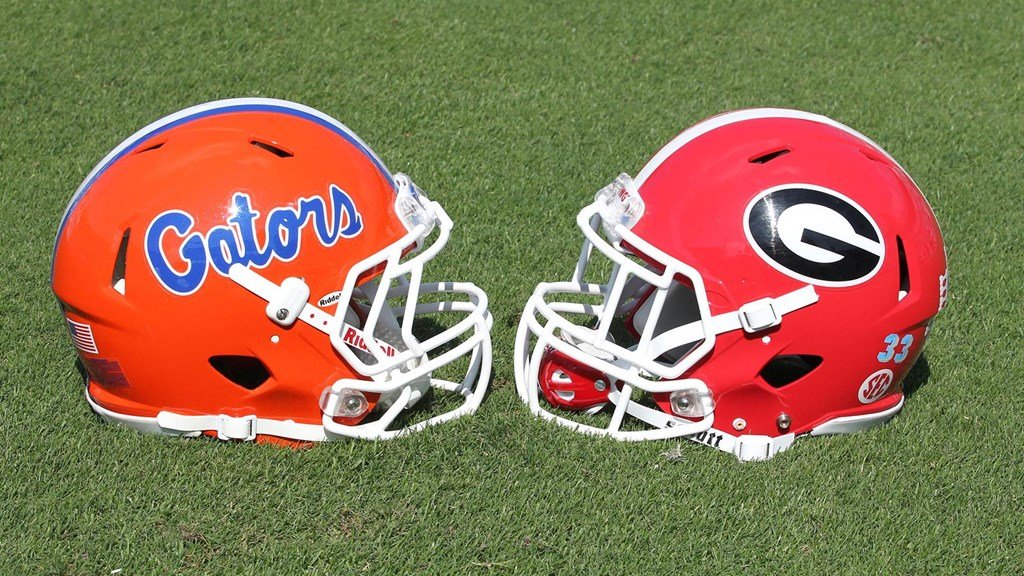This is a horizontally oriented photograph showcasing two college football helmets positioned face-to-face on a grassy field, which might be turf due to its even texture. The helmet on the left belongs to the Florida Gators. It stands out with its vivid orange color, featuring the word "Gators" in blue cursive outlined in white. The helmet also sports blue and white stripes running along its top, a white face mask, an orange and blue trim, and an American flag sticker on the back. The helmet on the right represents the Georgia Bulldogs. It is red with a striking black "G" inside a white oval, similar to the Green Bay Packers logo. The helmet has a white face mask, a red chin strap, a white stripe down the middle, and the number "33" on the back along with the SEC logo. Both helmets symbolize the storied rivalry of these SEC conference teams, captured in a close-up, dramatic, pre-game pose on the lush green field.